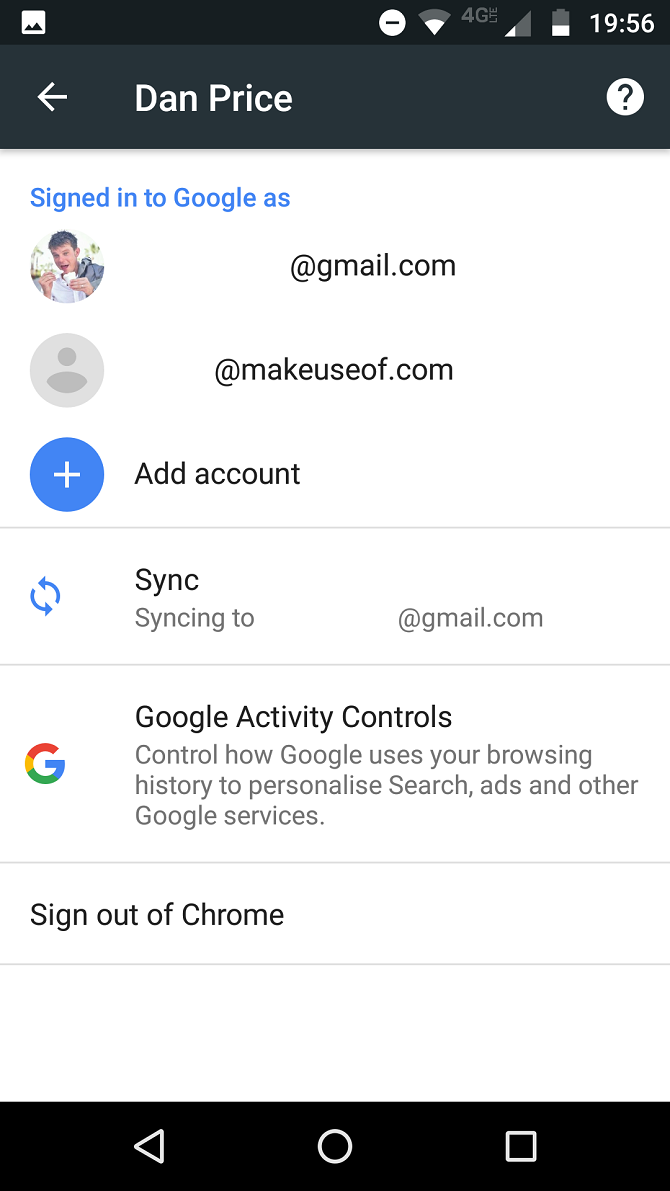The image depicts a screenshot of a smartphone's interface, likely from the settings or account management section related to Google services. 

At the top of the screen, there is a header bar with several icons indicating the status of the device: Wi-Fi signal bars, 4G connectivity, a half-full battery icon, and the time, which is shown as 19:56. The left side of the header features a back arrow, a name "Dan Price," and a black question mark inside a white circle.

Below the header, on a white background, the text "Signed in to Google" appears in blue. Underneath this text, there is a profile picture of a man with dark hair and a pale complexion, dressed in a grey outfit. He is eating something with a spoon from a styrofoam container, possibly ice cream. Next to the profile picture, his email address is shown ending with "@gmail.com".

Following this is another profile section, which is blank. It features a grey circle with a generic silhouette icon and an email address "blank@makeuseof.com". 

Next, there is a red and blue circle with a white plus sign and the text "Add account."

Continuing down the screen, there is a horizontal line dividing the sections. Below this line, there is a blue circle with two arrows forming a loop, next to the word "Sync." The text "sync to @gmail.com" follows this icon.

Below another dividing line, the Google logo (featuring red, yellow, green, and blue colors) is displayed with the text, "Google activity controls," followed by a description that reads, "Control how Google uses your browsing history to personalize search ads and other Google services."